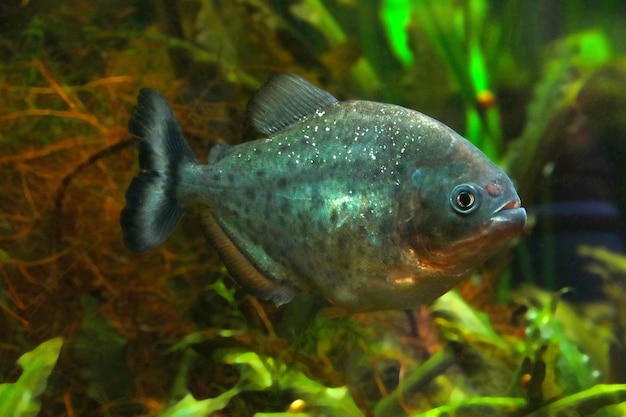The photograph captures a vibrant fish swimming in water, amidst a marshy, aquarium-like setting filled with a mix of brown, green, and orange vegetation. The fish, facing to the right, showcases a striking combination of colors: an emerald green body, a black and green face, and a bronze or gold underside. Its tail fin is black with a light vertical stripe in the middle, and it features small, visible fins with hues of dark blue and orange. The fish’s mouth is partially open, and its single visible eye is wide open, creating a sense of dynamic stillness against the backdrop of lush, artificial-looking reeds and grasses.